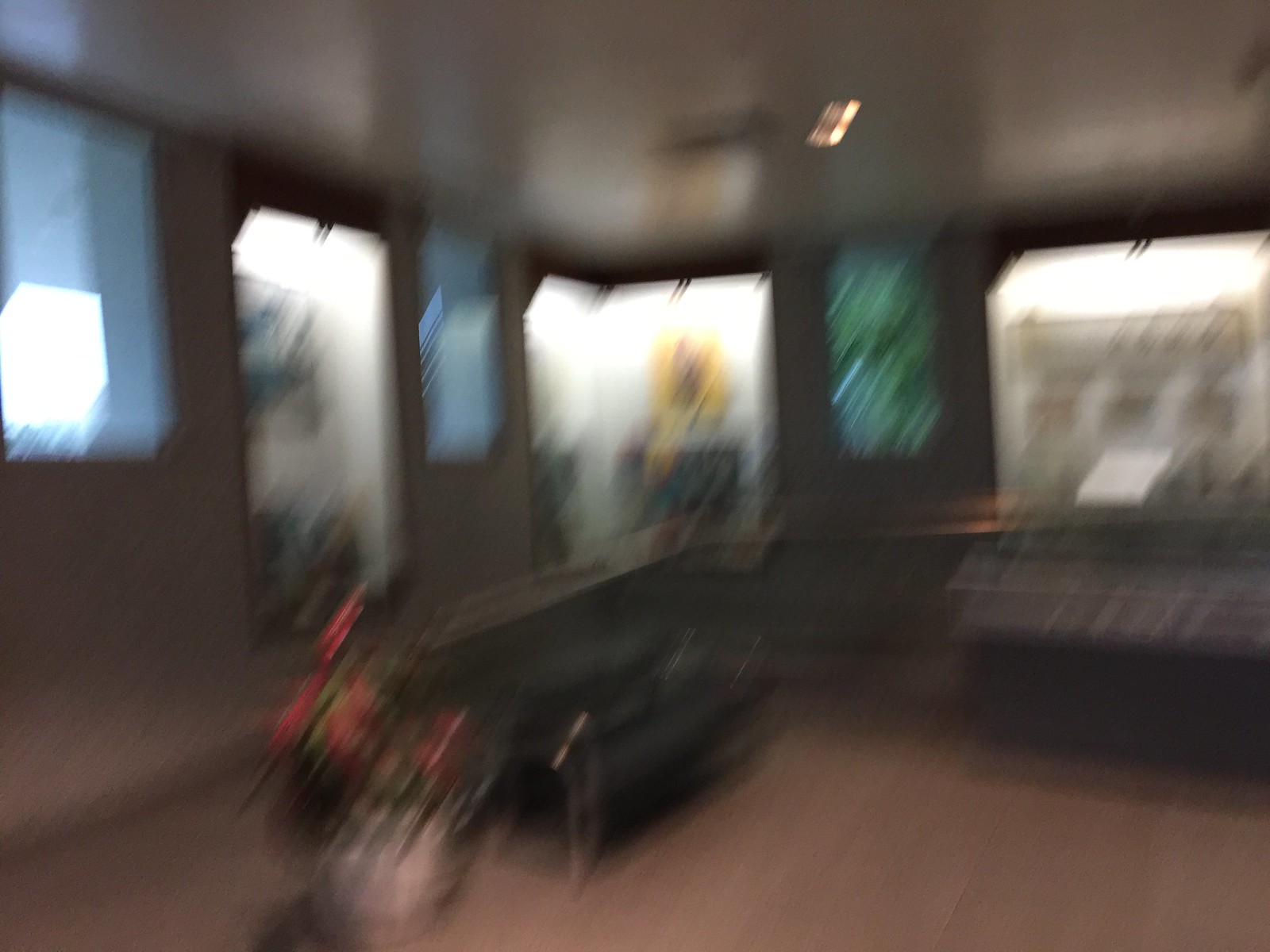A very blurry image depicts what appears to be a small room, possibly a museum or a tastefully decorated living space. The walls are lined with multiple display cases, some of which contain objects that are difficult to identify due to the blur. There's a notable array of glass cases housing various items, with three large and distinct pieces embedded in the wall, holding several mysterious objects. The ground is covered with a light brown carpet that extends to the walls, creating a warm and inviting atmosphere. 

In the center of the room, there is dark-colored furniture, including a two-seater couch on the middle left. Next to this couch is a vase full of roses, adding a touch of natural elegance. Additionally, a planter with flowers and greenery is visible on the left-hand side. 

The room also features a white ceiling and several light sources: a window on the left allows sunlight to stream through, accentuating the layout, and ceiling lights provide additional illumination. Notably, to the left of the window, there is a distinct planter or "spacer" with an emerald green color. Overall, although the image is quite fuzzy, it showcases a harmonious blend of decorative elements and display pieces, suggesting it might be an inviting private interior or an intimate museum space.